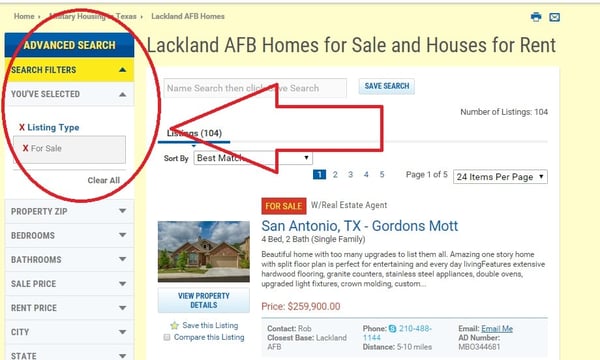A detailed description of the screenshot:

The screenshot captures a portion of a real estate website. At the top right corner, the website's title, "Lackland AFB Homes for Sale and Houses for Rent," is prominently displayed in black font. On the left side, there is a giant red-outlined arrow pointing towards the top left, accompanied by a label that reads, "Advanced Search: Search Filters You've Selected." Below this label, it specifies "Listing Type: For Sale," designating the properties being showcased.

On the bottom right of the screenshot, there is a default property listing. The listing is for a house located in San Antonio, Texas, identified as "Gordon's Mott." This house is available for sale, highlighted by an orange rectangle with "For Sale" inscribed within it. The listing mentions involvement with a real estate agent and details that it is a four-bedroom, two-bathroom single-family home. The description of the property reads: "Beautiful home with too many upgrades to list. Amazing one-story home with a split floor plan, perfect for entertaining and everyday living. Features extensive hardwood flooring, granite counters, stainless steel appliances, double ovens, upgraded light fixtures, and crown molding." The asking price for this home is $259,900, indicating it's ready for a new family to move in and start creating memories.